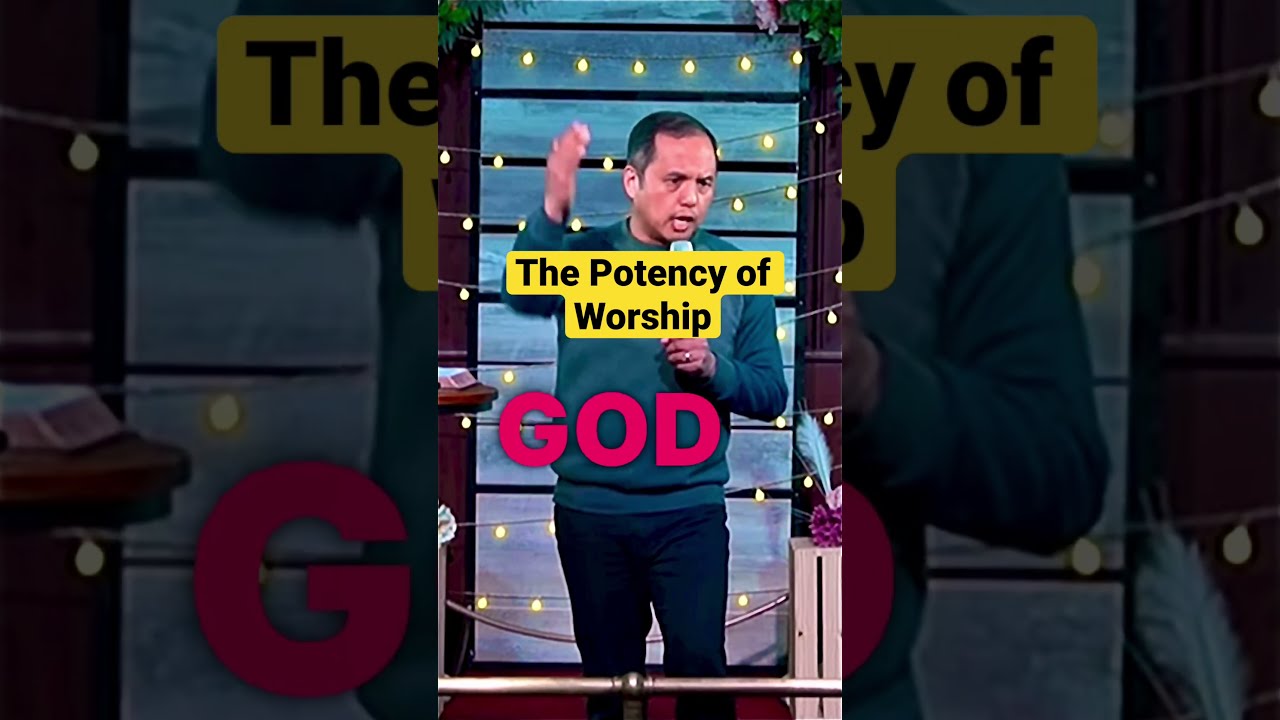In a horizontally rectangular image, split into three vertical panels, the central focus is on a man with short dark hair and olive-colored skin, speaking into a microphone held close to his mouth. He is dressed in a bluish-green sweater and black pants, gesturing with his extended right hand. The background features vertical wooden planks in shades of blue and violet, adorned with rows of small white string lights. Overlaid across the man's midsection is a yellow rectangle with the black text "The Potency of Worship," and below it in bold red letters is the word "God." The left and right panels are darker, displaying an enlarged and somewhat obscured continuation of the background and text, with segments of "The Potency of Worship" and "God" partially visible, alongside additional views of the strung lights and parts of the man’s figure.